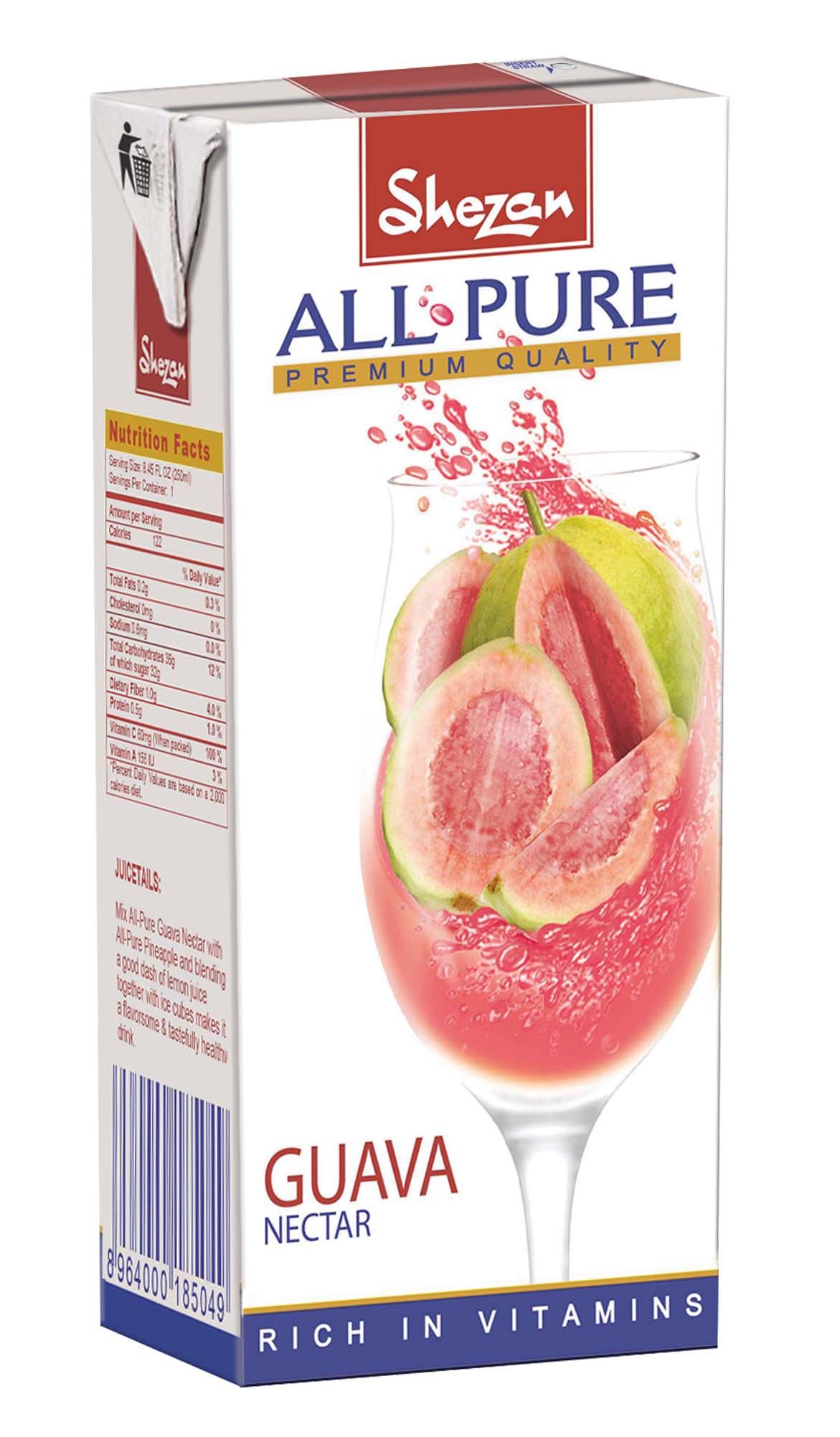The image features a rectangular box, prominently displaying the brand name "SHEZAN" at the top in white letters set against a red background. Below the brand name, there's a label that reads "All Pure" in blue, enclosed within a golden rectangle. Under this, there's a blue section with white text proclaiming "Premium Quality."

Central to the design, a transparent wine glass filled with pink guava juice is depicted, suggesting a refreshing beverage. Surrounding the glass, several ripe guavas are shown, adding a tropical vibe. The product name "Guava Nectar" is prominently displayed, with "Guava" written in bold red letters and "Nectar" in blue.

Towards the bottom of the box, the phrase "Rich in Vitamins" is printed in white letters against a blue background. Off to the side, near the lower edge, there is a serial number noticeable in blue. Additionally, a nutrition facts label is present, featuring a golden rectangle backdrop with "Nutrition Facts" highlighted in red.